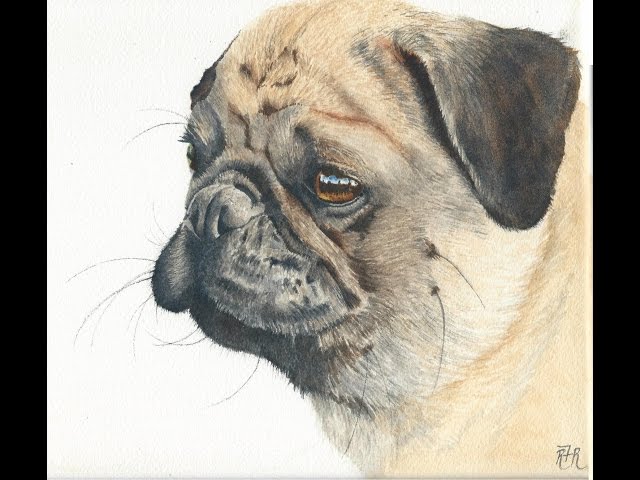The image is a detailed, color drawing of a pug mix dog's head, centrally positioned and looking towards the left. The dog's fur is a tan-gray color with black triangular floppy ears and various brown spots on its forehead. Black whiskers sprout from the sides of its short, stunted snout, and above its wet-looking, gold-colored eyes. The eyes are large and expressive. The nose is black and smooshed in, with black markings surrounding the nose, mouth, and extending between and under the eyes. The background is white, and the overall image is framed by black vertical borders on the right and left sides. In the bottom right corner of the drawing is the artist's signature, consisting of two capital "R"s. The image is clear and brightly lit, showcasing every intricate detail of the dog's face.